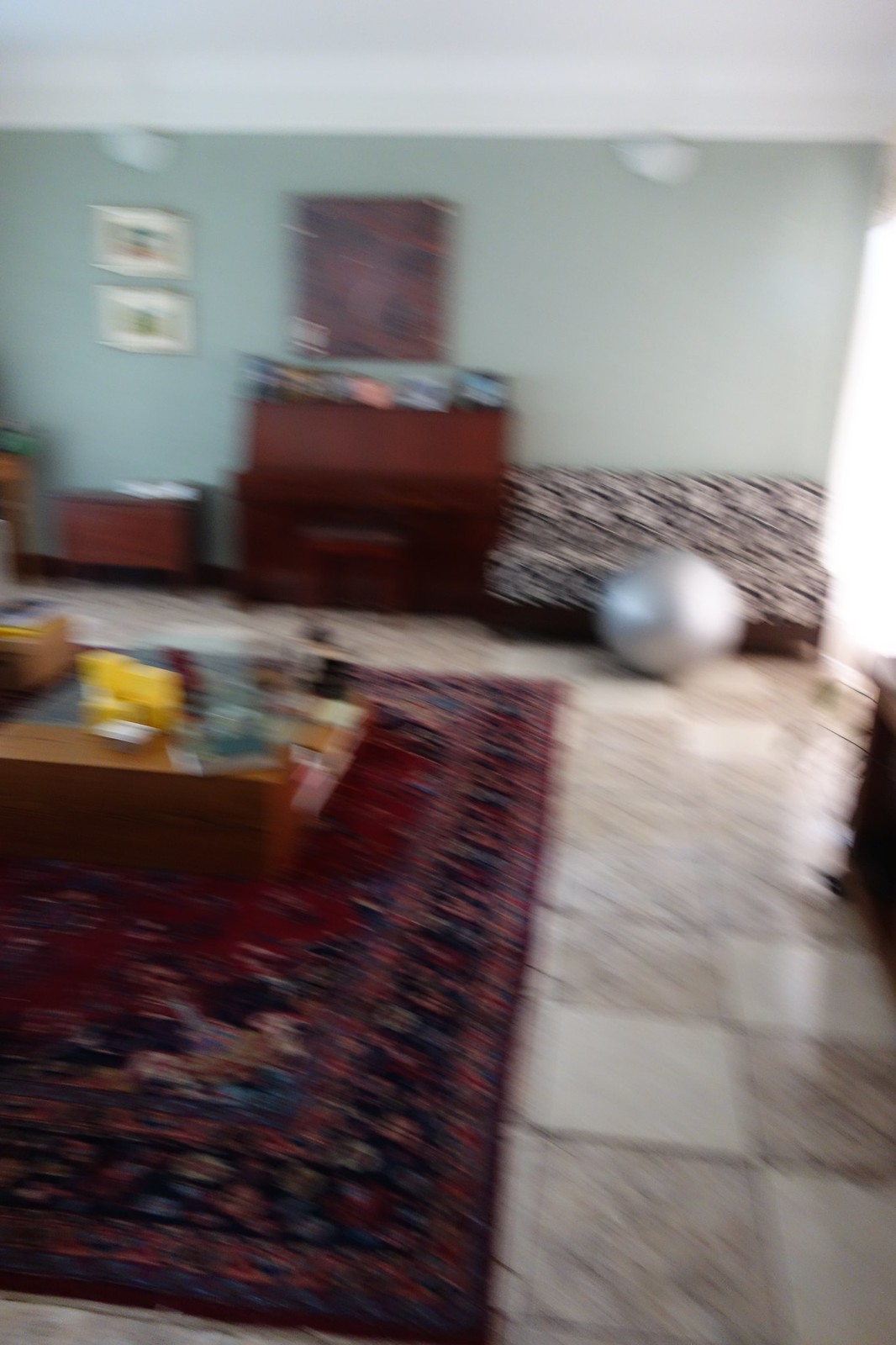A blurry color image captures the inside of a home living room that is painted in a light gray hue. The floor showcases a combination of brown and white checkerboard tiles on the right side, while a large dark red Turkish-style rug with intricate blue, red, and floral patterns occupies the center and extends to the left. Dominating the center of the room is a wooden coffee table cluttered with various indistinguishable items. On the right, a black and white couch is positioned against the gray wall, with a large silver exercise ball in front of it. Adjacent to the left of the couch is a dark brown stand-up piano accompanied by a small seat and adorned with picture frames on top. Above the piano hangs a large framed object, roughly half its width. Further to the left of the piano, a small wooden table sits against the wall, beneath two smaller pictures. Off to the far right corner, partially visible, is a likely TV stand, and beyond it, a brightly lit area hints at a window or a doorway leading to another room.